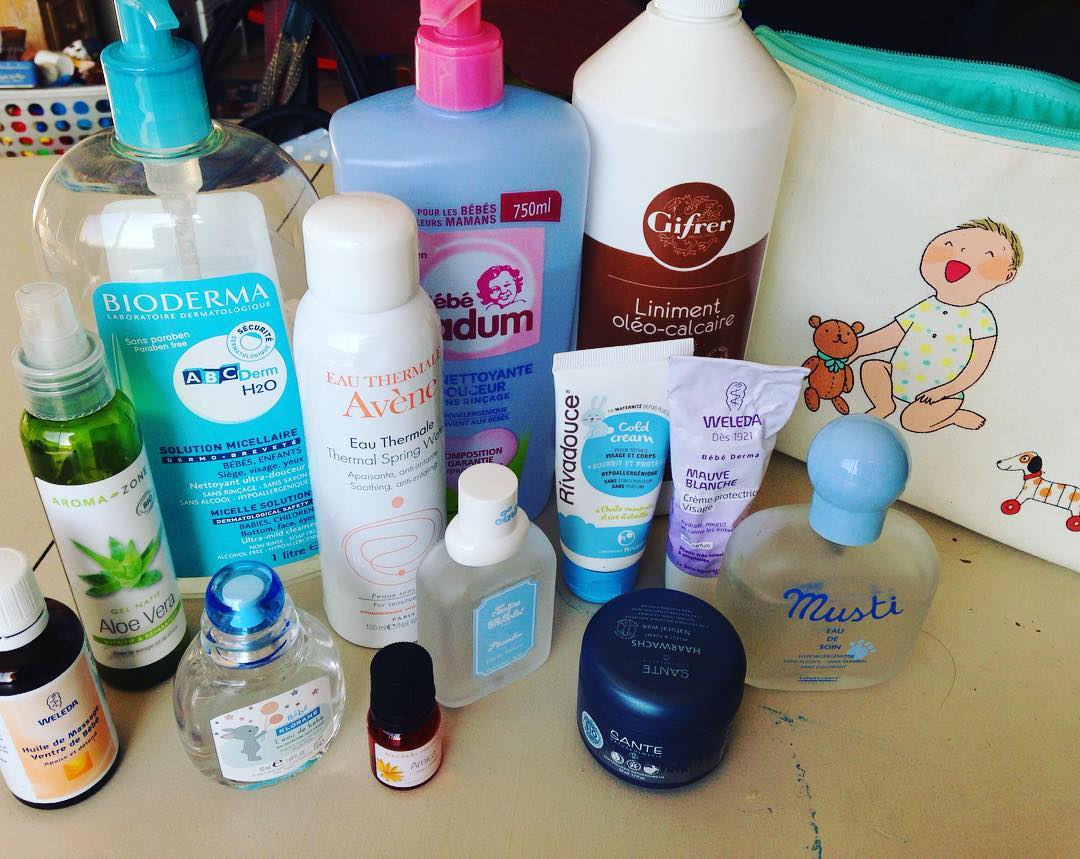The photograph captures an array of baby supplies and toiletries meticulously arranged on a white, concrete-like surface. From left to right, the collection includes:

- A small brown glass bottle with a white lid and a yellow label, though the text is not discernible.
- A taller green spray bottle equipped with a clear plastic spray top.
- A large clear plastic squirt bottle featuring a blue squirting top, labeled "Bioderma" in white on a blue label.
- A white metal canister with a white cap, inscribed with French text, including "Avene" and "Thermal Spring."
- A light blue lotion bottle with a pink cap and a gray label adorned with a little child's face.
- A large white bottle resembling a paint container, labeled "Liniment" in white on a brown label.

These items are neatly positioned in front of the camera, presenting a comprehensive view of various infant care products.